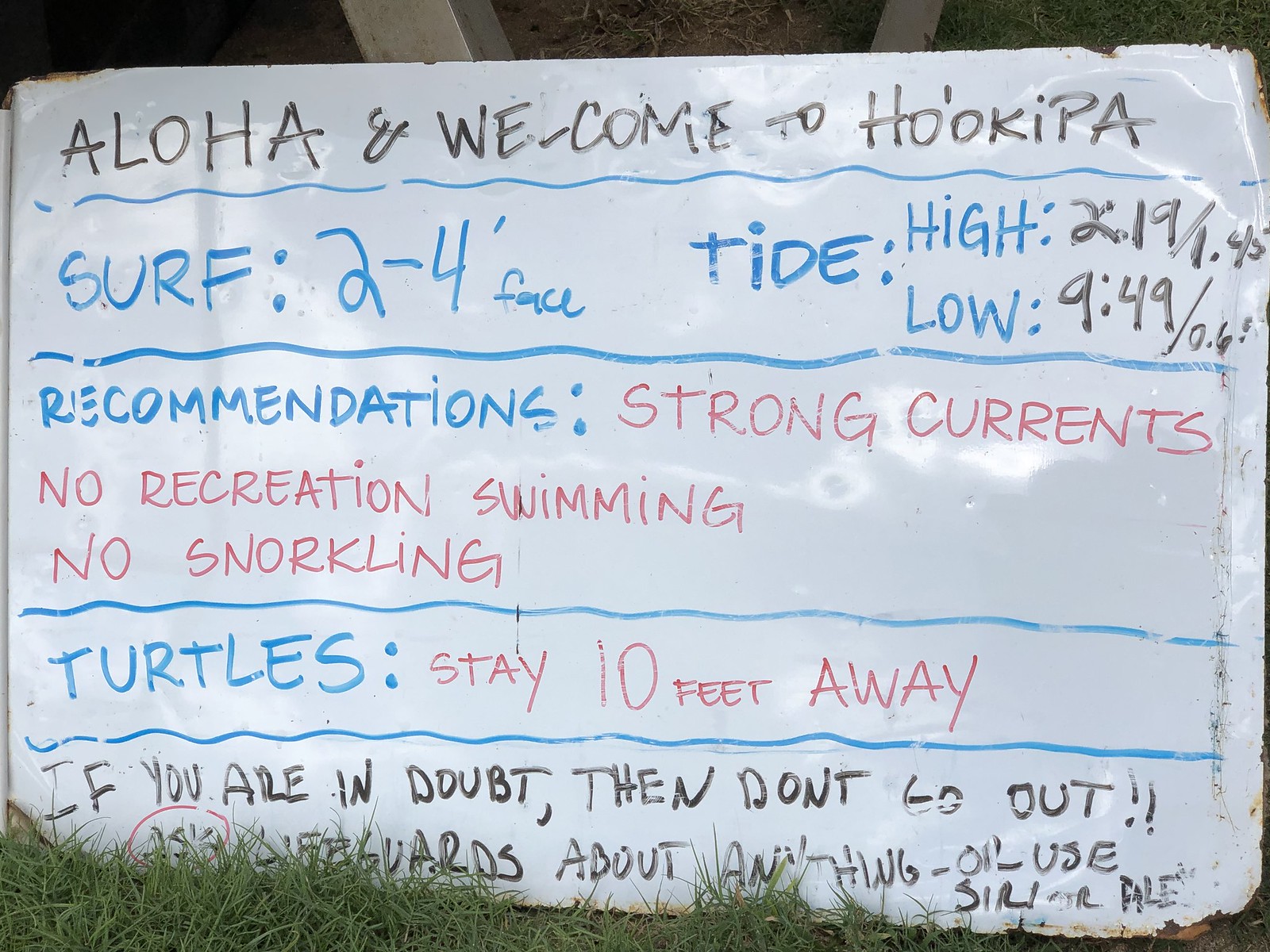This outdoor image displays a white dry erase board in an apparent state of disrepair, leaning against a metal frame with grass partially obstructing the lower portion. The board features announcements in both black, blue, and red letters. At the top, it reads "Aloha and welcome to Hookipa" (H-O-O-K-I-P-A) in black letters. Beneath this is a blue squiggly line, followed by blue text detailing surf conditions: "Surf: 2-4 inches face" and "Tide: high 219/145, low 949/0.65." Another blue squiggly line separates these details from further information. Blue text next reads "Recommendations:" to the right of which in red letters appear warnings: "strong currents," "no recreation," "swimming," and "no snorkeling." Additionally, there is a caution about turtles, advising to "stay 10 feet away." An important safety reminder reads, "If you are in doubt then don't go out." Some text at the bottom is obscured by grass and fading, but suggests consulting lifeguards for further assistance. The weathered edges and partially faded text testify to the board's aged condition.